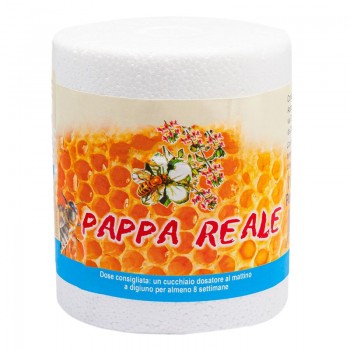This image features a cylindrical jar of honey with a white cap, positioned against a completely white background. Dominating the center of the jar is a tan-colored label adorned with various intricate details. The label prominently showcases an image of a honeycomb. Overlaying this honeycomb, there’s a striking display of flowers: a large white four-petal flower with a bee, possibly a yellow jacket, with its wings extended, hanging from it, and a red flower, likely a touch-me-not or four o'clock, with green stems and leaves. The words "PAPPA REALE" are displayed in bold red capital letters at the center of the label. In the bottom left corner of the label, another bee is depicted around white petals, enhancing the nature-inspired theme. A blue horizontal bar spans the bottom of the sticker, featuring white text, albeit not in English, adding a touch of international flair to the design.